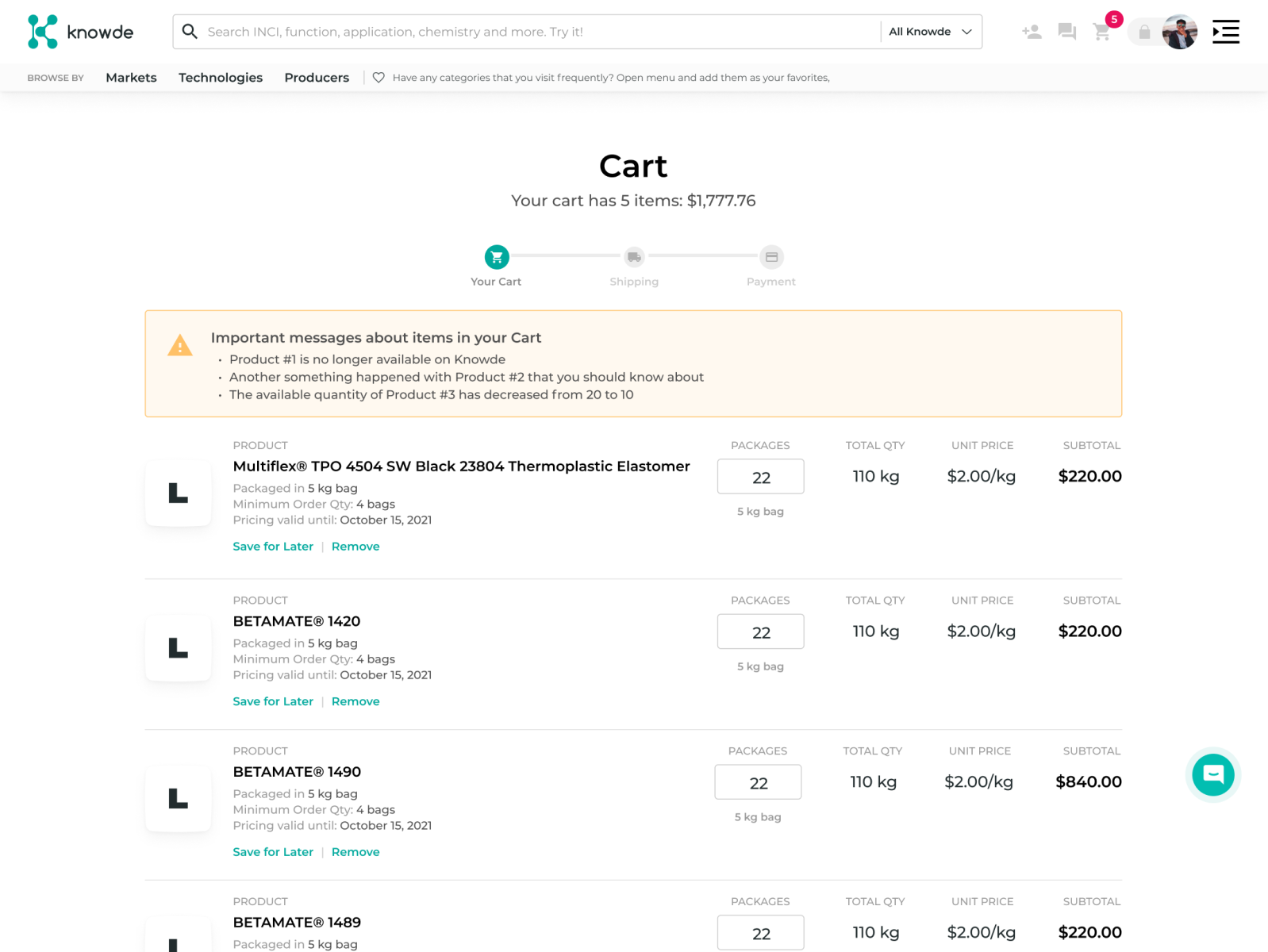**Detailed Captivating Caption:**

This image showcases the shopping cart summary page for Noti, an online shopping platform. At the top of the page, there's a distinctive header bar that includes several elements: 

1. **Brand Logo and Name**: Positioned at the top-left, the brand logo for Noti resembles a stylized "K" adorned with five green circles, indicating the company's identity. Adjacent to the logo is the text "Noti".

2. **Search Bar**: Centrally located in the header is a rectangular search bar with a magnifying glass icon, containing light gray placeholder text that reads "Search INCI, function, application, chemistry, and more. Try it." 

3. **Dropdown Menu**: To the right of the search bar, there's an 'All Noti' dropdown menu marked by a downward-facing arrow.

4. **User Icons**: Following the dropdown are several icons. These include a user icon with a plus sign, a chat icon, and a cart icon bearing a red or pink circle with the white number '5' inside it. There is also a lock icon next to a slider bar that displays a user avatar, potentially depicting an Asian young man on a beach background. Finally, there's a settings or information icon, which looks like two horizontal lines sandwiching a play arrow flanked with lines.

Beneath the header bar is a navigation menu with tabs that allow browsing by "Markets," "Technologies," "Producers," and "Favorites."

**Main Section - Cart Summary**:

5. **Cart Header**: The main body of the page features the cart summary. It begins with the word "Cart" and a statement, "Your cart has five items," followed by a total amount of $1,777.76.

6. **Checkout Process**: The checkout process is divided into three steps, visually represented as icons: "Your Cart" in green with accompanying grey text, followed by "Shipping" and "Payments" in grey.

7. **Important Messages**: A warning box displayed with a yellow boundary and light yellow fill contains a warning triangle icon and the alert message highlighting important updates concerning items in the cart:
   - Product 1 is no longer available.
   - A pertinent issue with Product 2.
   - Availability of Product 3 has decreased from 20 units to 10.

**Cart Details**:

8. **Item Rows**: The cart displays four rows, each detailing a product:
   - **Icon and Description**: Each row begins with an 'L' shaped icon within a rounded corner white box, followed by the product name, a fine text description including packaging details, minimum order quantities, and the validity dates of the pricing.
   - **Actions**: Options to save for later or remove an item are available, marked in teal green.

9. **Package and Quantity**: The subsequent columns list the number of packages (each product has 22), total quantity (each product totals 110 kg), unit price (each item is priced at $2.00 per kg), and subtotal amounts ($220, $220, $840, and $220 respectively for the four products).

10. **Communication Icon**: A teal chat bubble icon with a white messaging bubble inside it is situated to the far right of the third product row, suggesting a communication option related to this item.

This detailed and comprehensive layout ensures that users can efficiently manage their shopping experience with Noti.